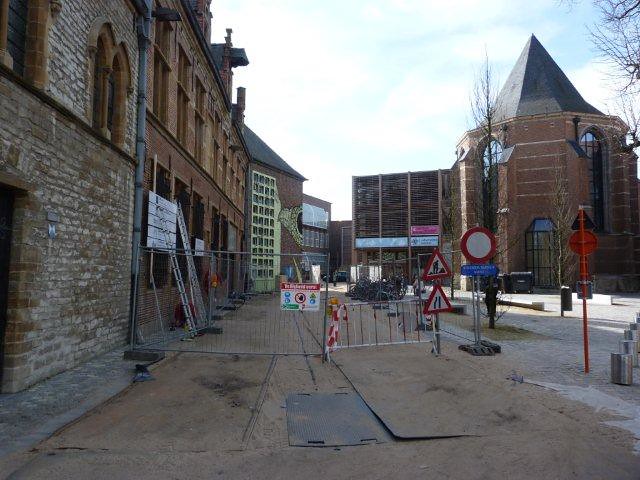This photograph captures an urban area undergoing construction or potentially condemned. Prominently, large brick buildings surround the scene on both the left and right sides. The building on the right features a distinct, almost triangular, gray roof, adding a unique architectural element to the photo. The ground within the fenced-off area appears to be covered with a material resembling cardboard, and there are multiple construction signs, including a red stop sign and another indicating work in progress. Additionally, metal debris litters the blocked-off road, indicating it's unsafe for travel. Snow patches on the right side suggest a colder day, and the leafless trees further confirm the wintery setting under a partly cloudy blue sky. The overall scene is devoid of people, emphasizing the restricted access and ongoing work in the area.